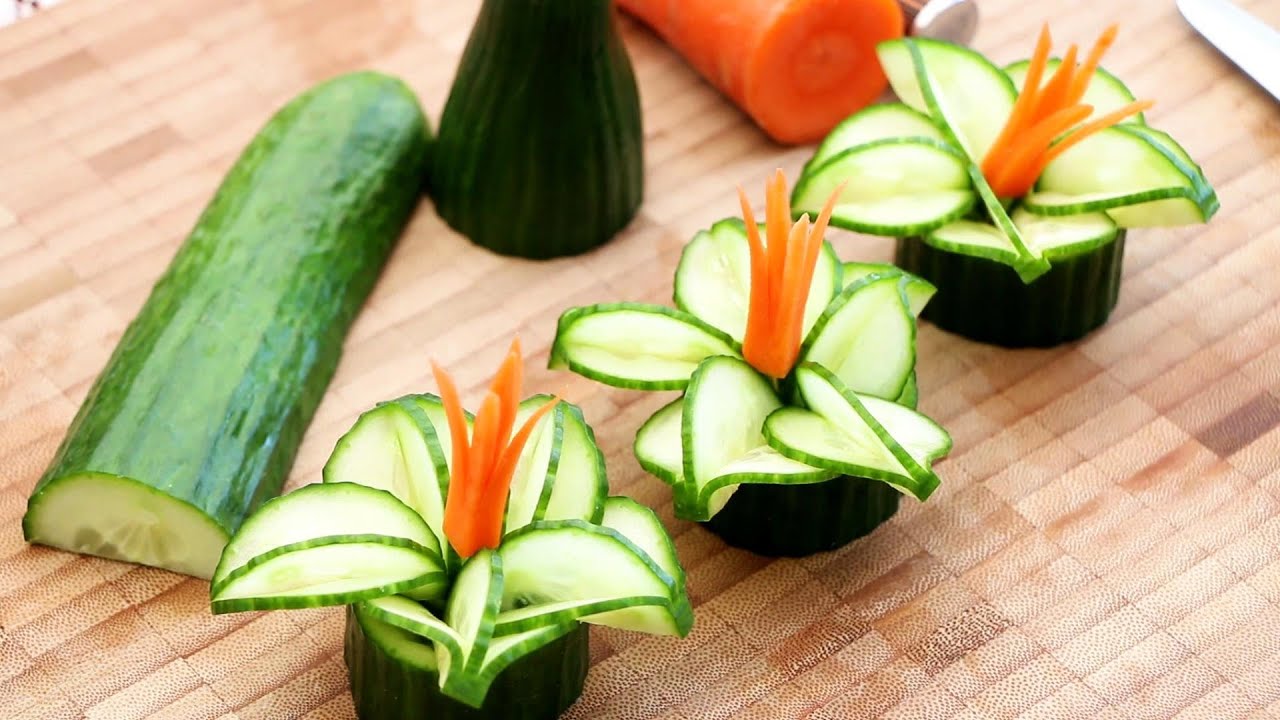This image showcases an artistic arrangement of sliced cucumbers and carrots, designed to mimic floral patterns. Delicately thin cucumber slices, organized with green edges, form the petals of these vegetable "flowers." At their centers, vibrant orange carrot pieces protrude, completing the floral illusion. These intricate decorations are placed in small black containers positioned on a cabinet composed of small, rectangular wooden pieces. On the left side of the image, a half cucumber, cut through the middle, rests flat, exposing its rounded top and green skin. Additionally, a partially visible carrot and the tip of a knife can be spotted in the photograph, which is rectangular and oriented longer than it is tall. The overall scene highlights the creativity in transforming simple vegetables into elegant decorations.